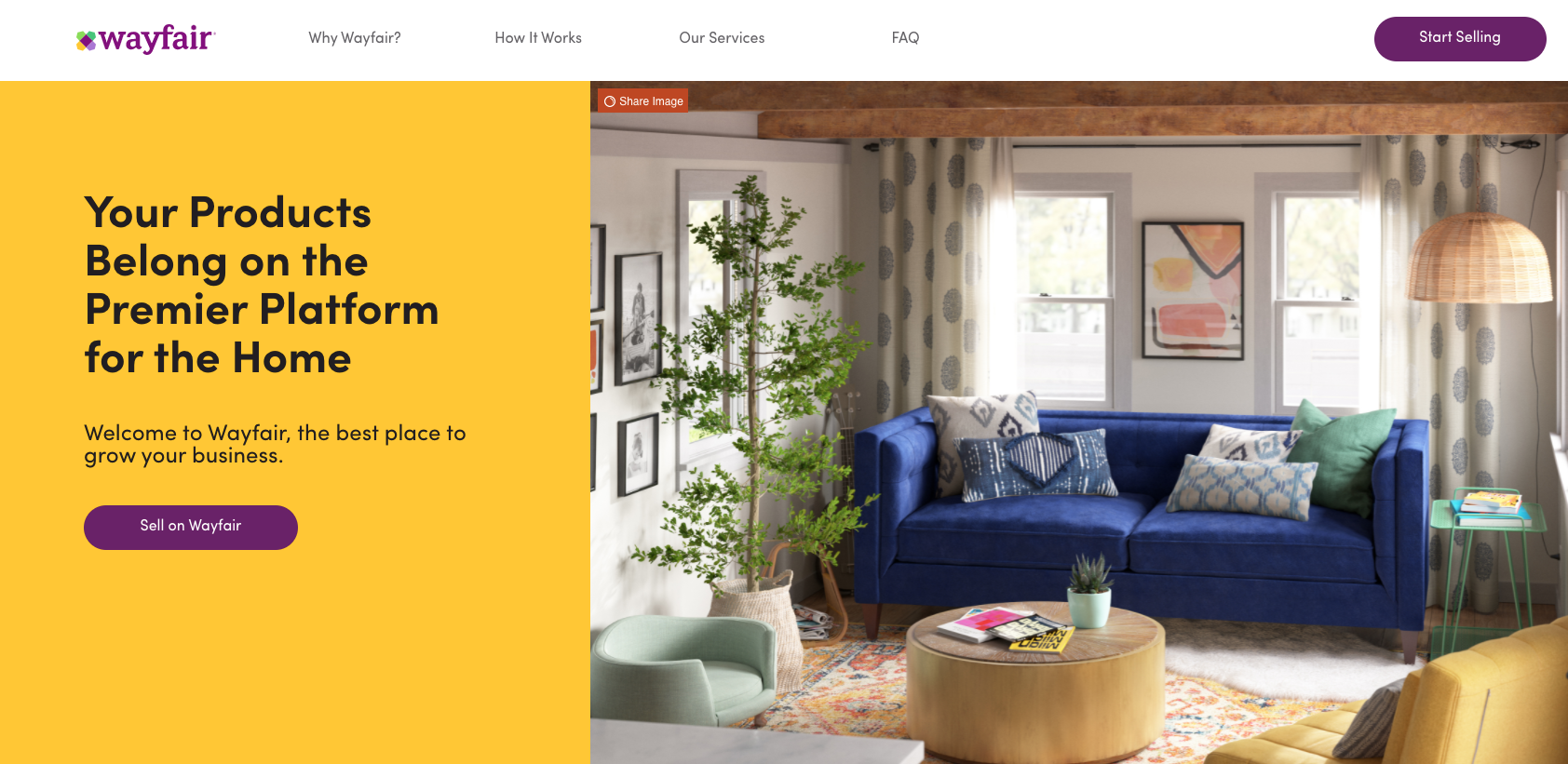The image displays the Wayfair home website interface. In the top left corner, the Wayfair logo is prominently featured, accompanied by the Wayfair icon. Adjacent to the logo, a white space transitions into a section labeled "Why Wayfair?" in grey text, followed by a question mark. Next to this, there are links to "How it Works," "Our Services," and "FAQ." Moving to the top right, there's a "Start Selling" button, adorned with white font and set against a striking purple, bubbly background.

Beneath this header, a vibrant yellow banner is situated on the left side of the screen, with bold black text stating, "Your products belong on the premier platform for the home. Welcome to Wayfair, the best place to grow your business." Below this message, another "Sell on Wayfair" button is found, echoing the earlier design with white font against a purple, bubbly bar.

On the right side of the screen, an inviting image of a modern living room is depicted. This room features a blue sofa adorned with five distinct pillows, each showcasing varying designs such as triangles and horizontal stripes in blueprints. Among these, one pillow is green. A circular coffee table stands in front of the sofa, topped with a lush plant, adding a touch of nature to the cozy and stylish living space.